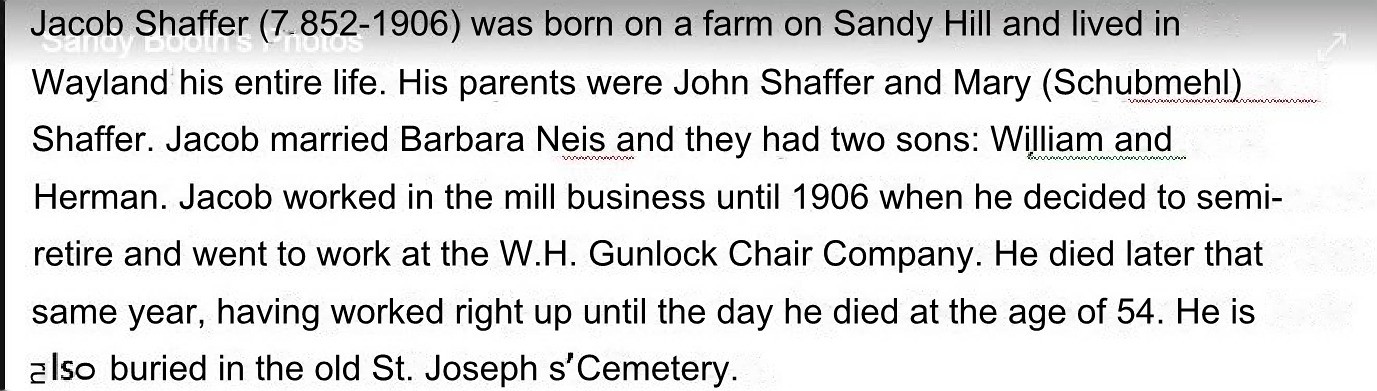The image shows a screen capture of a Word document featuring an obituary paragraph. The prominently black text on a white background recounts the life of Jacob Sarver (incorrectly noted as Jacob Shaffer in some parts), born on a farm on Sandy Hill and residing in Wayland his entire life. His parents were John Sarver and Mary (Scooby or Schubmehl) Sarver. Jacob married Barbara Diaz and they had two sons, Colin (reported by one person), William, and Herman. Jacob worked in the mill business until 1906 when he semi-retired and joined the W. H. Gunlock Chair Company. Tragically, he passed away the same year at the age of 54, having worked up until his death. He is buried in the old St. Joseph's Cemetery. The text is concisely edited and highlighted with underlining typical of Microsoft Word's spell checker, indicating a typical screen capture format.